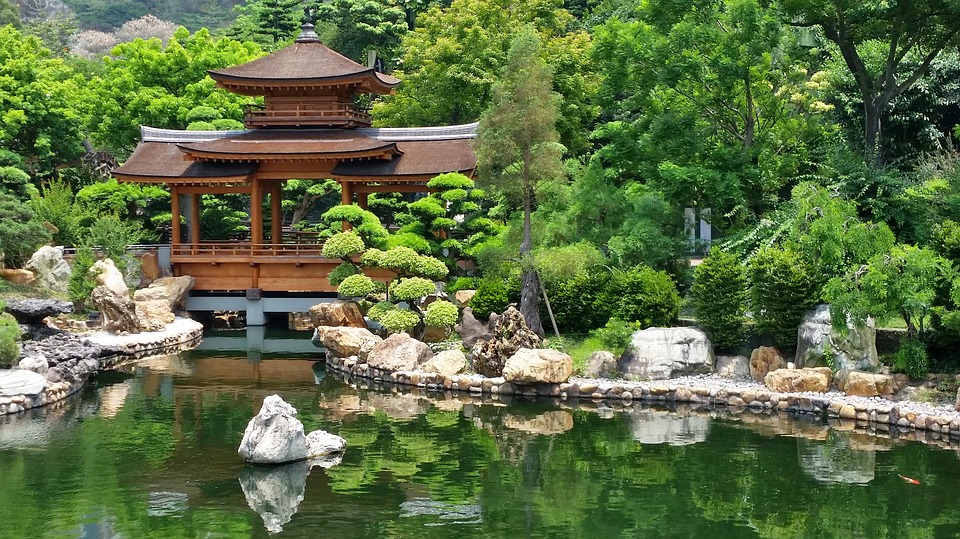The image depicts a picturesque Japanese garden set against a backdrop of lush, vibrant, and dense forestry. Central to the scene is a large wooden pagoda with a distinctive tiered, curved roof featuring black and silver detailing, sitting on a gray platform that anchors into the water. The pagoda extends over a wooden bridge with metal supports underneath. A serene pond, reflecting the green of the surrounding trees, stretches across the foreground, populated by koi fish. The scene is accentuated by man-made landscaping, including a stone walkway, large gray and brown rocks, and bonsai trees that delicately frame the water's edge. Towards the background, a heavily forested mountain looms, enhancing the garden's natural beauty and tranquility. The entire setting exudes an atmosphere of calm and serene beauty, epitomizing traditional Japanese garden aesthetics.